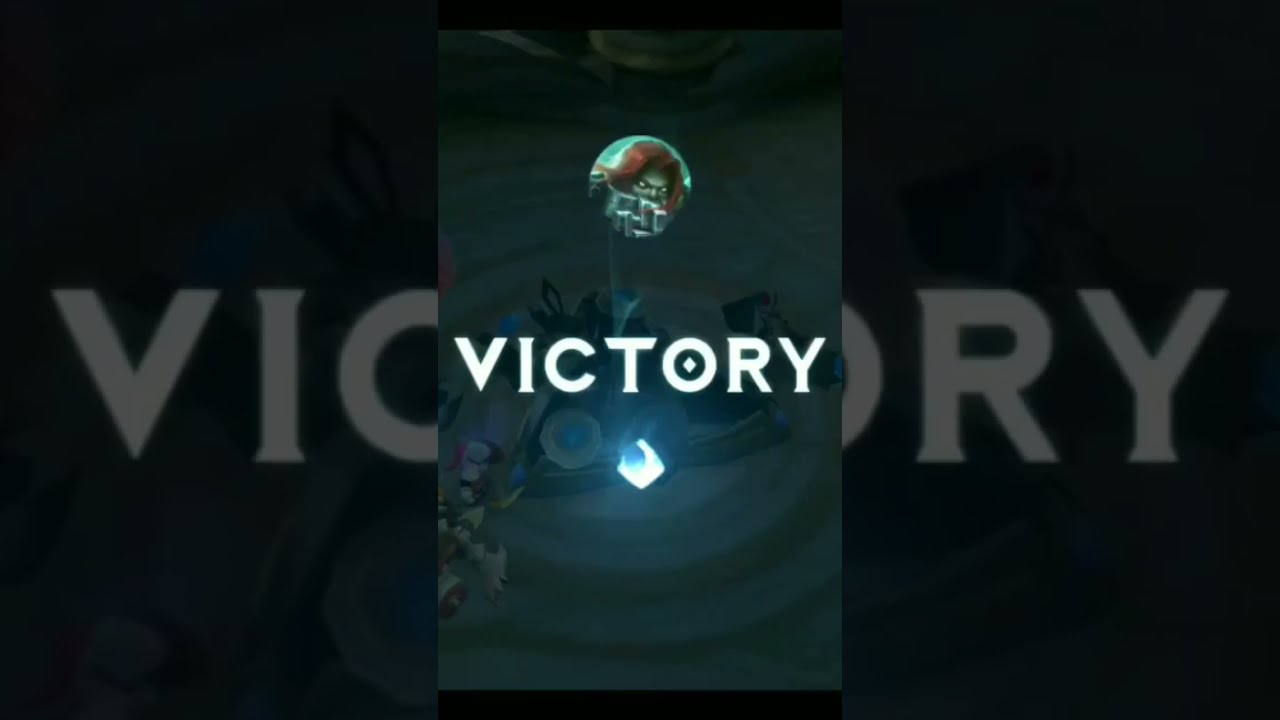The image is a tall rectangular section, likely a screenshot from a game’s victory screen. Dominating the center of the image is the word "VICTORY" in bold, white uppercase letters, slightly glowing blue. Below this text, a glowing blue diamond shape is present, adding to the ethereal atmosphere of the victory announcement.

Above the word "VICTORY," a circular overlay reveals the upper part of a malevolent-looking character. This character has strikingly bright red hair, yellow eyes without pupils, and green skin. The character’s gaze is intense and directed toward the viewer, suggesting a sense of triumph or dominance. This figure is likely adorned in heavy armor, contributing to an imposing presence.

The background of the image is dimmed to highlight the victory elements. It displays a scene reminiscent of a base, with repeated circular lines and possibly sandy terrain. Additional visual elements include a spiral on the ground and blurred structures within triangular shapes, adding complexity to the background.

Enclosing the main content, the left and right sides of the image are bordered by grayed-out, enlarged segments of the central design, creating a seamless yet distinctive frame. The overall composition emphasizes the triumph and intensity of the moment.